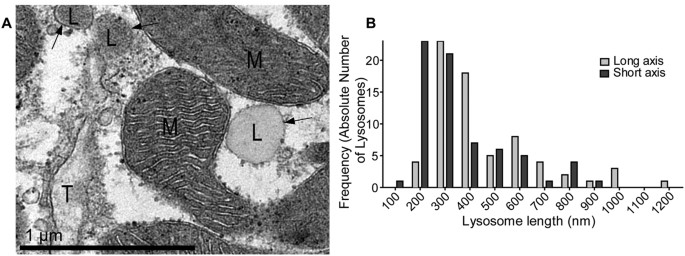The black-and-white image comprises two distinct sections labeled A and B. Section A, situated on the left side, features a detailed drawing representing a microscopic view of microorganisms of varying shapes and sizes. The drawing includes several labeled cells: light grey circular shapes denoted with the letter L, larger, darker grey oval and teardrop shapes marked with the letter M, and a long, skinny shape at the bottom left labeled T. These cells are rendered in different shades of grey, providing contrast and aiding in differentiation. To the right of this drawing in Section A, a bar graph is present. This graph compares the frequency (absolute number of lysosomes) to lysosome length, measured in micrometers (M). It includes numbers along the left axis indicating frequency (0, 5, 10, 15, 20) and along the bottom axis showing length (ranging from 100 to 1200 M). At the top right of the graph, a legend identifies a long axis represented by a grey square and a short axis by a black square. The entire image, devoid of color, uses varying shades of grey for clarity and emphasis.